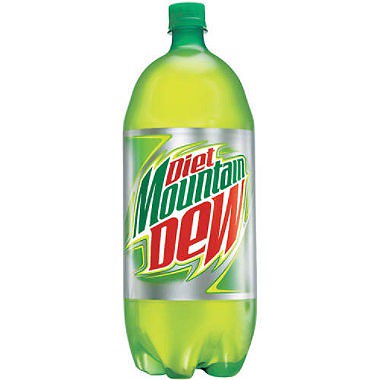The image features a two-liter bottle of Diet Mountain Dew, prominently characterized by its classic green hue and medium green cap. The bottle appears to be full and unopened, with the iconic label design clearly visible. The label showcases a vintage logo from the mid-2000s, with "Diet" and "Dew" in red text, while "Mountain" is in a darker green, all set against a silver background with green accents. The lighting creates a slightly darker edge around the bottle, emphasizing its contours. The background of the image is a plain white, highlighting the bottle as the primary focal point.